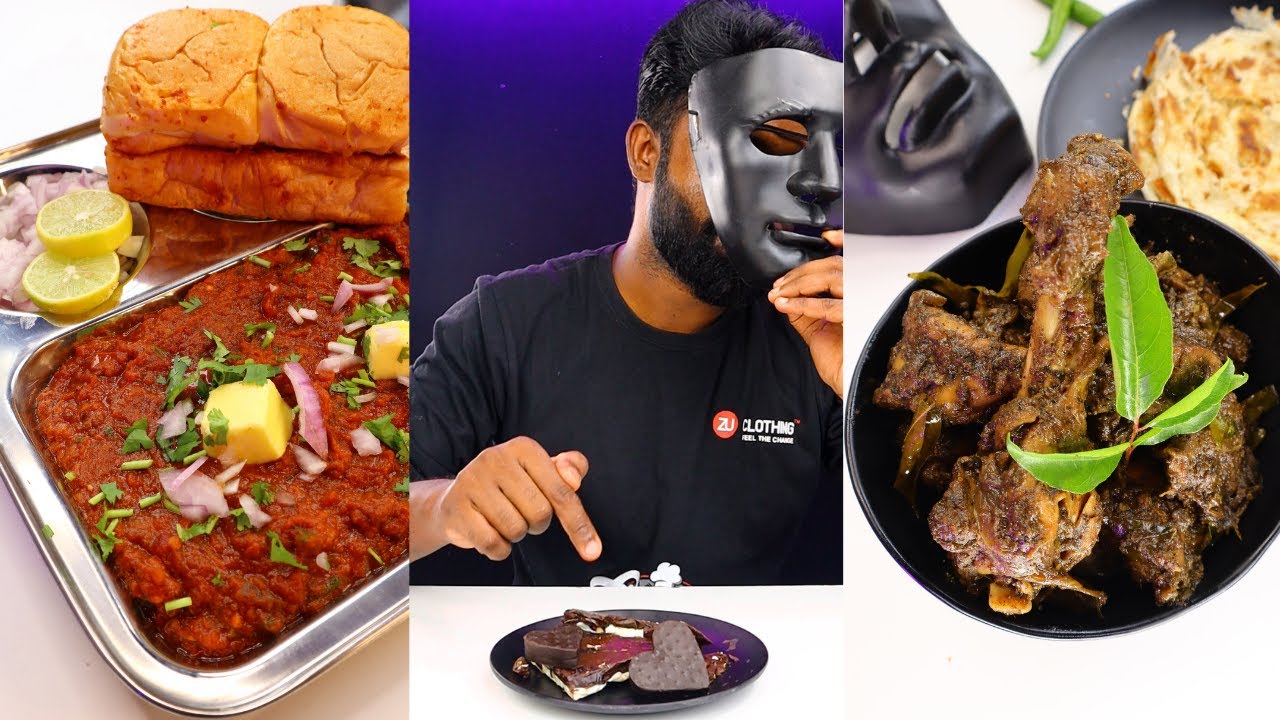This composite image features three vertically aligned photographs like a triptych, each crammed with intricate details centering around a taste-testing event. The left photo, taken from above, showcases a diverse spread: a pan of lasagna drenched in tomato sauce and adorned with chopped parsley, red onion, and melting squares of butter. Nearby, a loaf of freshly baked bread sits enticingly, flanked by a dish containing chopped onions and two lemon slices.

The central photograph captures a man with black hair and a full beard, dressed in a black shirt with "ZU" branding in orange and white lettering. He is captured mid-action, removing a silver mask, and pointing down at a black plate containing large chocolate hearts wrapped in golden foil.

On the right, another detailed scene is presented. A black bowl houses grilled beef garnished with a leafy sprig, accompanied by a background bowl containing browned mashed potatoes. Overlapping this scene, the edge of the previously seen silver mask is noticeable, adding coherence to the collage. Predominant hues of red, black, and brown unify this richly detailed composite, creating a vivid narrative of gastronomic exploration.